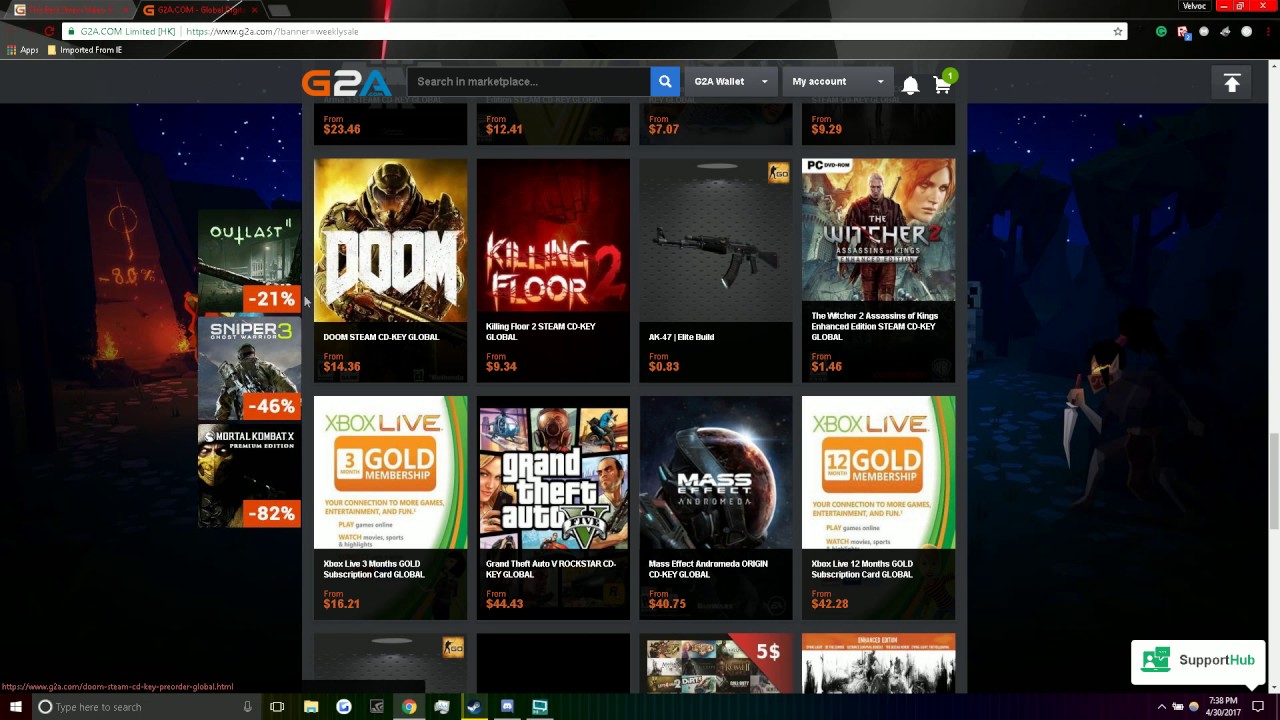The image features a detailed display of video game purchases from the digital marketplace G2A. Prominently shown is a variety of games available for purchase. At the center is "The Witcher," listed as PC compatible, which requires user login and wallet access, indicated by the 'My Assure' label. The shopping cart contains one item. 

Below, several highlighted titles include "Doom," "Killing Floor 2," and an indistinguishable game with an automatic weapon on its cover. "The Witcher" is also prominently displayed, followed by an "Xbox Live 3 Month Gold Membership." Adjacent to this is "Grand Theft Auto" and "Mass Street." Additionally, there is an option for an "Xbox Live 12 Month Gold Membership." 

To the left of the main display are three smaller, discounted games: "Outlast" with a 21% discount, "Sniper 3" at 46% off, and "Martial Chemetics" reduced by 82%. The display showcases the variety and savings available to gamers.